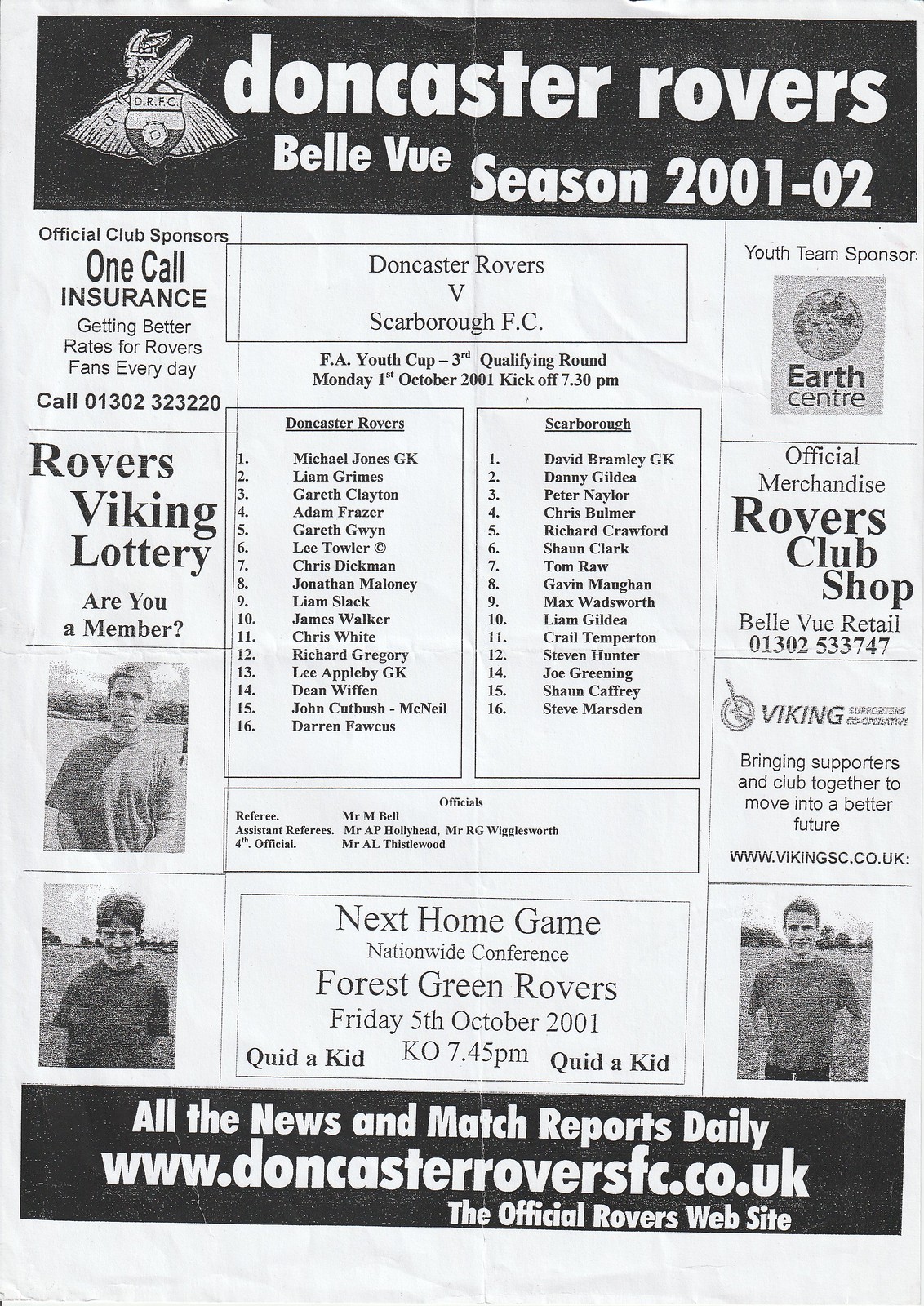A black and white image depicts a scanned poster for the Doncaster Rovers football team, highlighting their 2001-2002 season. At the top, within a black rectangle, it reads "Doncaster Rovers Bellevue Season 2001-2002" and prominently features the Doncaster Rovers logo (DRFC) to the left. The poster announces an upcoming match between Doncaster Rovers and Scarborough FC, listing the names of 16 players for each team in two separate squares. The left side and right side of the flyer showcase various sponsors and advertisements, including "Official Club Sponsors OneCall Insurance, getting better rates for Rovers fans every day" with a phone number provided. Additionally, the bottom of the flyer mentions "Official Merchandise Rovers Club Shop" and lists Earth Center as the youth team sponsor. It features some blurred pictures of football players. For news and match reports, it directs readers to the official Rovers website at www.doncasterroversfc.co.uk. The overall appearance suggests it might have been circulated as a newspaper insert.